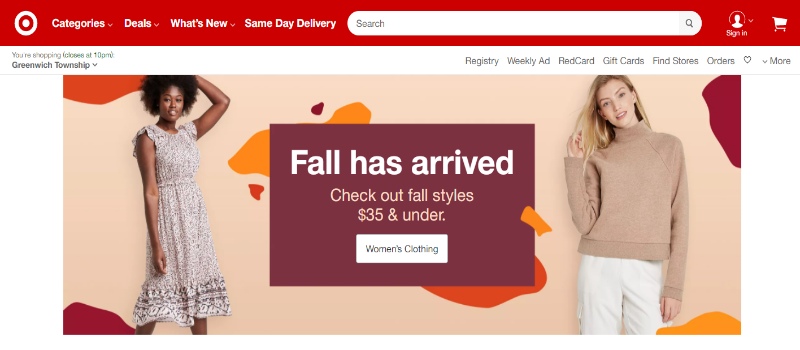This image is a detailed screen capture of a Target website. At the top, a distinct red bar houses the recognizable white Target bullseye logo, which is flanked by several submenu options in white: Categories, Deals, What’s New, Same Day Delivery, followed by a search box featuring a magnifying glass icon and the word "search." Adjacent to this, a red-and-white icon prompts users to sign in, and a white cart icon signifies the shopping cart.

Immediately below, text indicates the local store closing time, situated in Greenwich Township, which is paired with additional submenus: Registry, Weekly Ad, RedCard, Gift Cards, Find Stores, Orders (accompanied by a heart icon), and More.

Dominating the page is an image set against a tan background with splashes of orange, gold, and burgundy. The focus is on two models: an African-American young woman with curly black hair, wearing a brown floral-patterned dress, posed with one hand behind her head; and a Caucasian woman with blonde hair, clad in a tan sweater and white pants, seen twirling a lock of her hair.

Centered between the models, a burgundy box announces in white text: "Fall has arrived. Check out fall styles, $35 and under," accompanied by a clickable box labeled "Women's Clothing." The image stands out for its clarity and the ease with which all elements are readable.